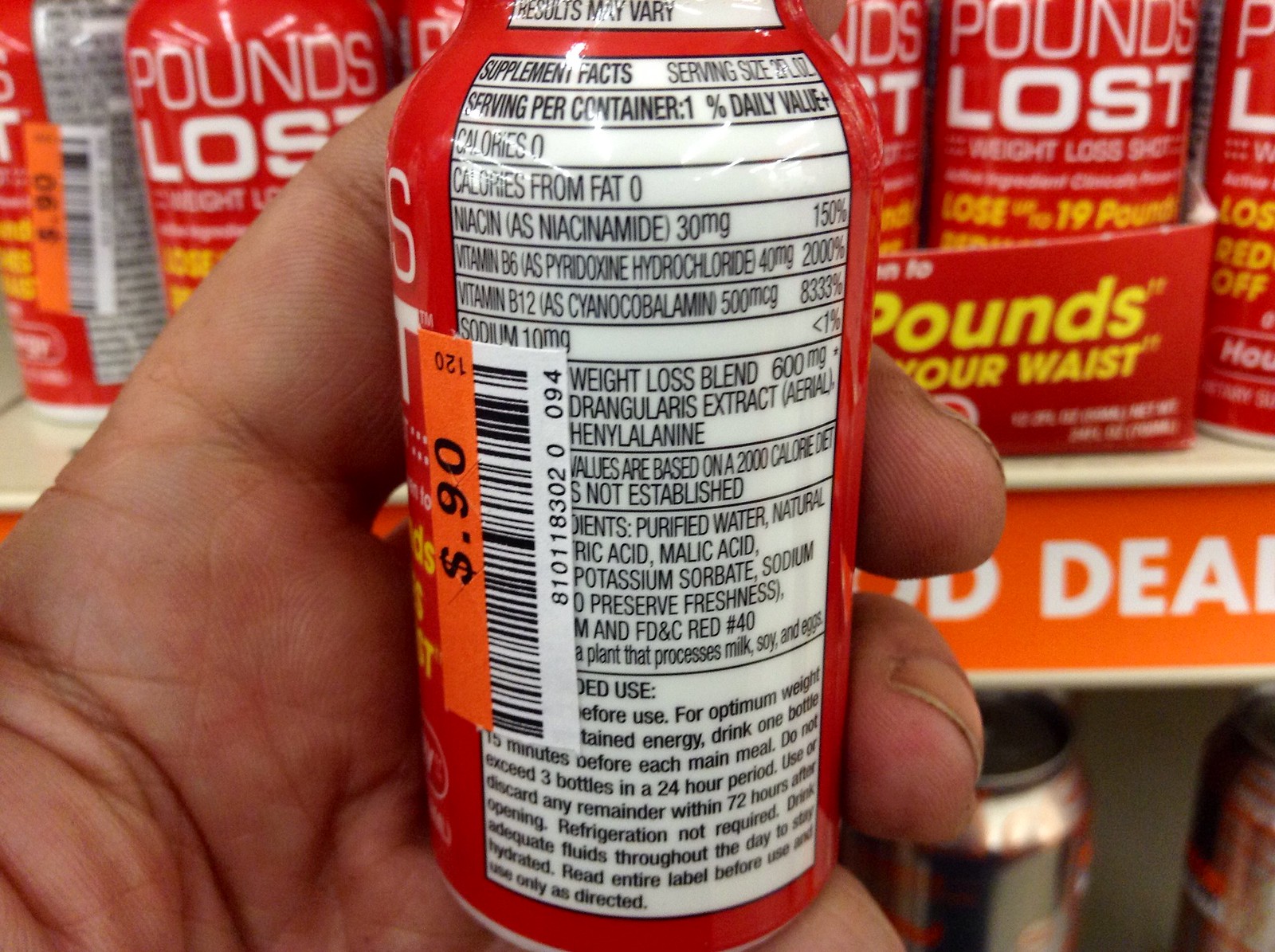A close-up image shows a person's left hand, fingers partially visible and fingernails notably dirty, holding a red and white plastic bottle prominently labeled for weight loss. The bottle features an orange 90-cent price sticker and detailed nutritional information on its back, including values for Niacin, Vitamin B6, Vitamin B12, Sodium, and a proprietary weight loss blend. The label also carries warnings and usage instructions, detailing serving size, safety precautions, and storage recommendations. Positioned in front of shelves, the bottle is part of a display where numerous identical bottles can be seen inside a red cardboard box with yellow writing. Above this main display, an orange "deal" sticker is only partially visible, and further up, additional bottles and two metal cans occupy the shelves.